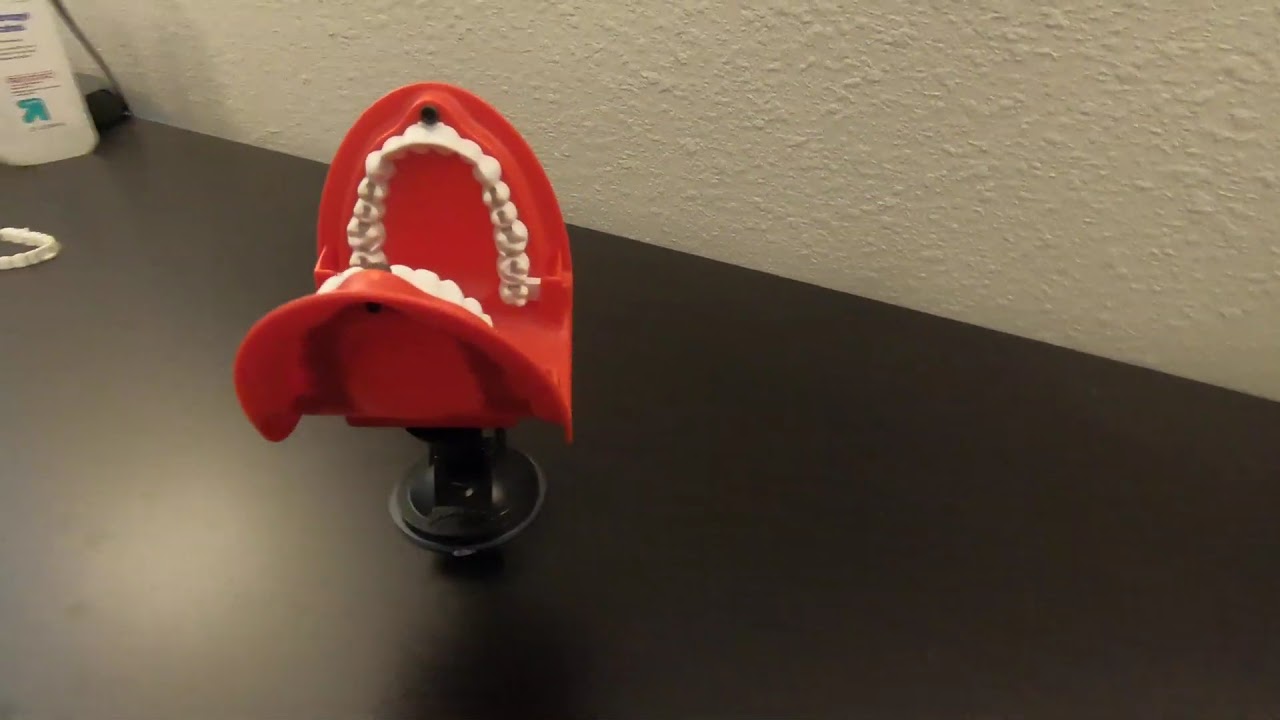This image depicts a detailed, lifelike dental model placed on a grayish-black desk. The model, featuring a pinkish-red gum with plastic white teeth, is oriented upwards, as if the mouth is opening towards the ceiling. The base is a dark, plastic material. Behind the model, a textured white wall serves as the backdrop. To the left of the dental model, there is another set of plastic teeth positioned on the desk. Additionally, a bottle with an indistinct blue logo is also situated on the table. In the top left corner, a pamphlet or display with a turquoise arrow and blue and black text leans against a small metal bar or plaque.